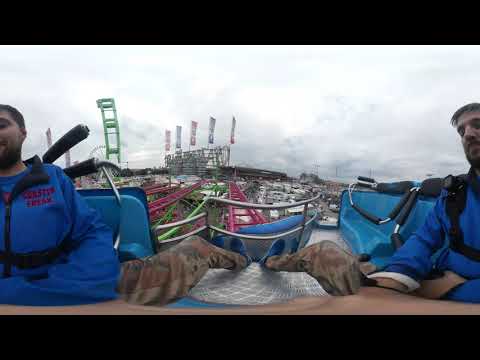In this photograph, two men are captured on an amusement park ride. They are high in the air, both wearing bright blue shirts with black safety harnesses, and are seated in blue seats on opposite sides of a large open ride structure. Behind them, the scene unfolds with various roller coaster tracks in vibrant colors—blue, pink, and green—along with a large green bridge-type structure and several flag-topped structures adding to the festive atmosphere. The ground beneath the ride features a distinct silver flooring. The sky above is heavily overcast, casting a gray, cloudy light over the entire setting, adding a sense of dramatic tension to the image. The photograph appears to have a fisheye lens effect, which somewhat distorts the scene, enhancing the dynamic and exhilarating atmosphere of the amusement park.